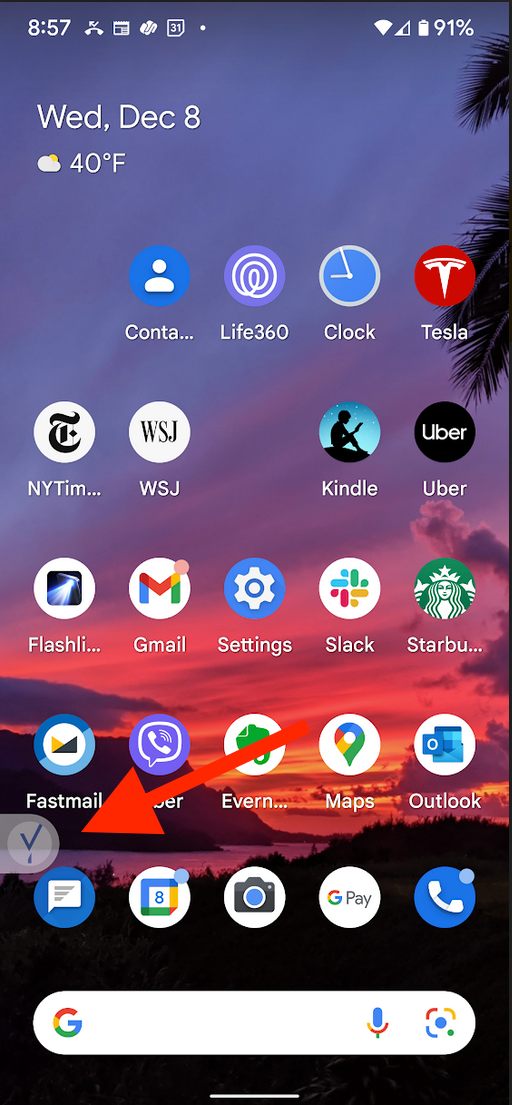The image is a detailed screenshot of a mobile phone home screen. The background features a picturesque photograph of a volcanic island, shrouded in silhouetted greenery. In the top right corner, the fronds of a palm tree are silhouetted against a bright sky. The sky itself is vibrant, showcasing a gradient that transitions from orange at the lower right to pink clouds, then to thick pink and purple clouds in the center, and finally to a lavender-blue hue at the upper left.

At the top of the screen, white icons are located on the left and right sides. Below, aligned to the left, white text reads "Wednesday, December 8th." Directly underneath, a simple light gray cloud icon with a gold sun peeking from behind it denotes the weather, accompanied by the text "40°F."

Dominating the bottom of the screen, a white, pill-shaped search bar is superimposed on the black silhouette background of the volcanic island. On the left end of the search bar, there's a multicolored "G" logo representing Google. To the right, it features a multicolored microphone icon, followed by a multicolored Google Lens icon. The Lens icon has three distinct corners: the top left is red, the top right is yellow, the bottom left is blue, along with a large blue circle in the center and a small blue circle on the bottom right.

Finally, towards the very bottom of the screen, a thin white line stretches horizontally across the center. Slightly above and to the left of this line, a translucent gray tab with a rounded right side is visible. Within this tab, a translucent white circle houses a distinctive black "Y" shape. A prominent red arrow points upwards from the right side, drawing attention to this tab.